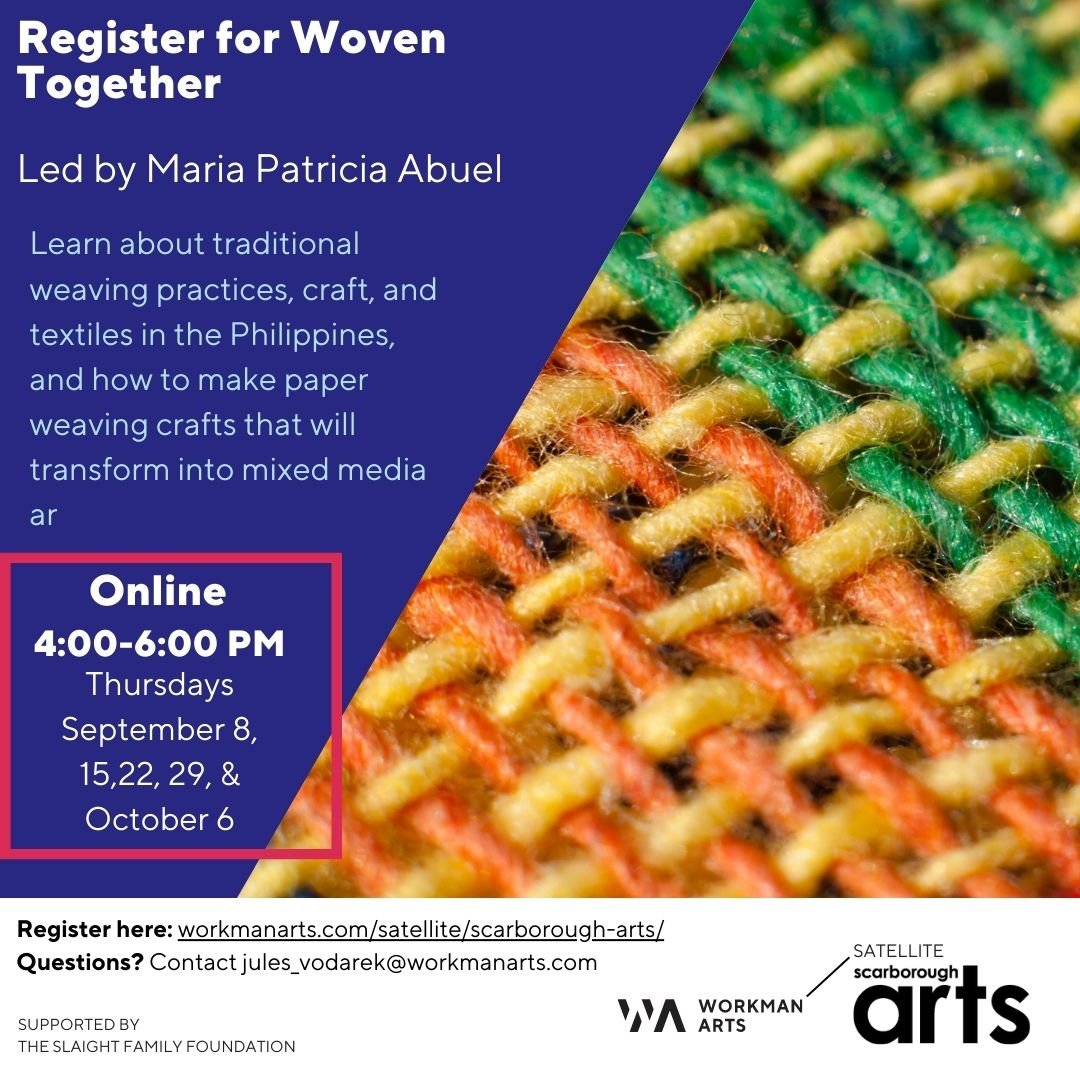The informational poster, sponsored by Satellite Scarabard Arts and Workman Arts with support from the Slate Family Foundation, is promoting a weaving workshop titled "Woven Together," led by Maria Patricia Abuel. The poster is square-shaped and split diagonally in the middle. On the right side, an up-close view of fabric shows a woven texture with green, yellow, and orange threads. The left side, in a blue section with white text, announces: "Register for Woven Together, led by Maria Patricia Abuel. Learn about traditional weaving practices, craft, and textiles in the Philippines, and how to make paper weaving crafts that will transform into mixed-media AR." Below this, a red box with additional details states that the sessions are held online from 4 to 6 p.m. on Thursdays: September 8, 15, 22, 29, and October 6. Instructions for registration are provided with a link: workmanarts.com/satellite/scarabard-arts/. For any questions, contact Julius The Dark at workmanarts.com. Emblems for Workman Arts and Satellite Scarborough Arts are also displayed, symbolizing their support and association with the event.